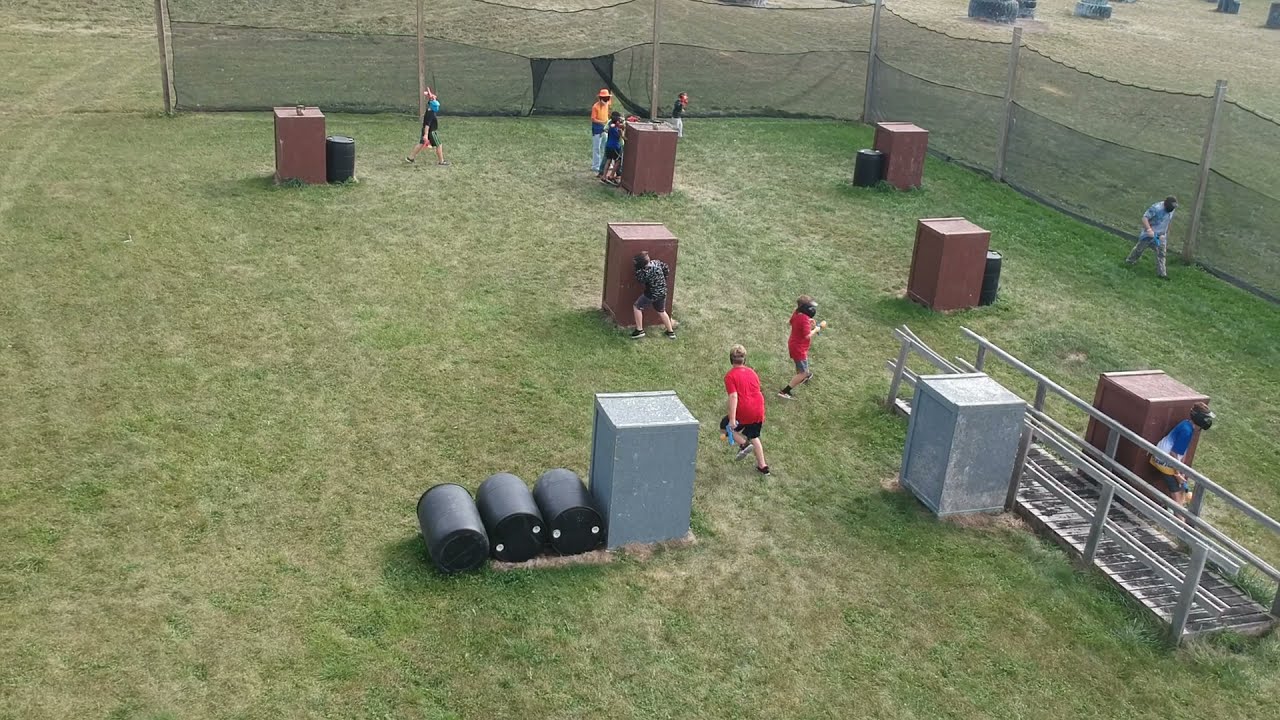In an outdoor paintball field set against a backdrop of lush green grass, various wooden and metallic crates are scattered around, creating a complex obstacle course. Encircled by a high netted fence, the field features several tubular walkways and a few black barrels positioned at the bottom of the image. The scene is bustling with activity, as eight people of varied ages, some in bright orange t-shirts and others in camouflage outfits, partake in a spirited paintball match. Many participants are equipped with headgear and paintball guns, taking cover behind the tall, rectangular wooden crates scattered throughout the field. One individual can be seen crouching behind a crate while another peeks out from behind another, hinting at the intensity of the game. The mix of colors—shades of green, black, gray, red, blue, tan, and orange—adds vibrancy to the scene, set in what appears to be a sunlit day, suggesting perfect conditions for this thrilling outdoor event.